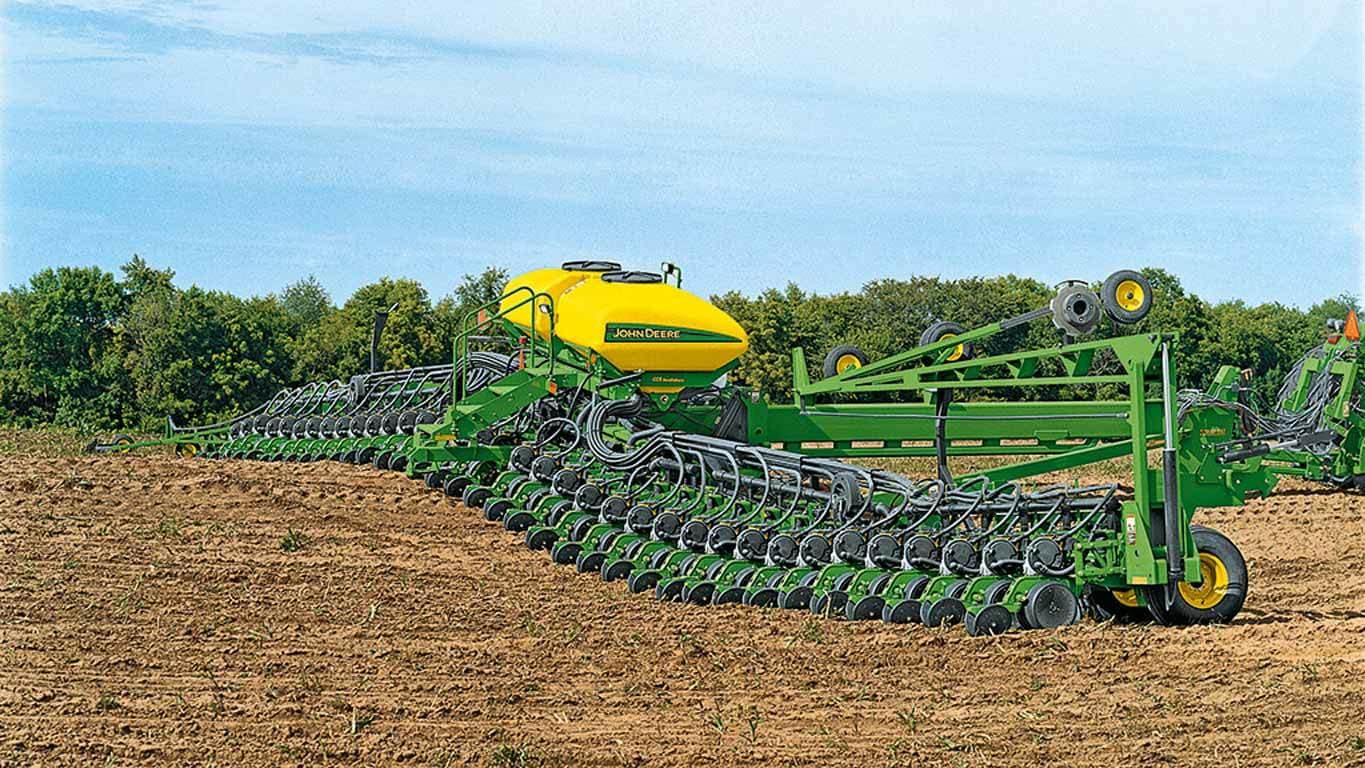This image showcases a vast field with an impressive piece of John Deere farming machinery spanning almost the entire width of the terrain. The machinery is unmistakably John Deere, painted in the brand's iconic green and yellow colors, and features the recognizable logo. Dominating the center are two large yellow tanks, likely used for storing water or other agricultural necessities. This substantial equipment, equipped with numerous wheels, hints at its specialized function, perhaps as a tiller or plow, designed to work the soil or water crops. The mechanism includes circular, V-shaped plow elements meant to dig into the earth, assisting in crop cultivation. In the foreground, stairs lead up to the central yellow tanks, suggesting ease of access for maintenance or operation. The freshly planted field is predominantly dirt-colored with no visible crops yet. The backdrop consists of a row of green deciduous trees under a clear, bright blue sky, indicating the season is likely early summer. On the right side of the image, the rear end of a green John Deere tractor is visible, indicating it may be towing the large farm apparatus across the field.